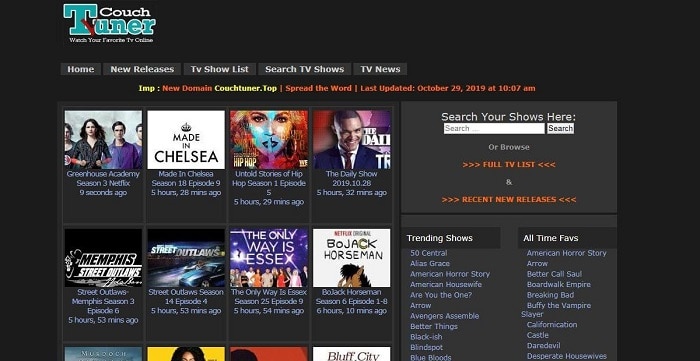The image is a screenshot of a website named CouchTuner, speculated to be a platform for streaming TV shows. The header of the website has a black background, with the word "Couch" displayed in white and "Tuner" in a teal color. Below the title, there are navigation options including "Home," "New Releases," "TV Show List," "Search TV Shows," and "TV Shows."

Beneath the navigation bar, there's a notification text saying, "New domain: CouchTuner Top. Spread the word. Last updated October 29, 2019, at 10:07 am." The main section of the page showcases eight featured TV shows, arranged in two rows of four.

The top row includes:
1. A show titled "Academy" in the upper left.
2. "Made in Chelsea."
3. "United States of Hip Hop Season 1."
4. "The Daily Show."

The bottom row features:
1. "Streets of Memphis Outlaws."
2. "Street Outlaws Season 14, Episode 4."
3. "The Only Way is Essex."
4. "BoJack Horseman."

On the right side of the screen, there is a search bar labeled "Search TV Shows Here," along with sections listing "Trending Shows" and "All-Time Favorites."